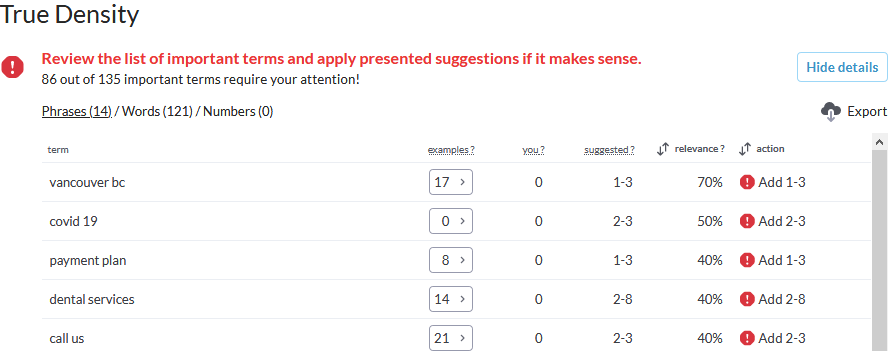The image displays a detailed notification screen against a white background. In the top left corner, the title "True Density" is prominently featured in bold black text, with both "T" and "D" capitalized. Directly below the title, there is a noticeable red stop sign icon with a white exclamation mark inside. Following this icon, in bold red text, it states: "Review the list of important terms and apply presented suggestions if it makes sense."

Further down, in black text, it is mentioned that "86 out of 135 important terms require your attention," followed by another exclamation mark. To the far right, there is a blue-outlined box with a white background containing the blue-text option "Hide Details." Beneath this, there is a cloud icon with an arrow pointing downwards, labeled "Export" with a capital "E."

Moving back to the left side, the screen categorizes the data into different sections:
- "Phrases (14)"
- "Words (121)"
- "Numbers (0)"

The data is organized into a table with six columns labeled as "Term," "Examples," "You," "Suggested," "Relevance," and "Action."

The rows of the table detail various terms as follows:

1. **Vancouver, British Columbia**
   - Examples: 17
   - You: 0
   - Suggested: 1 to 3
   - Relevance: 70%
   - Action: Add 1 to 3 (with a circular exclamation point icon)

2. **COVID-19**
   - Examples: 0
   - You: 0
   - Suggested: 2 to 3
   - Relevance: 50%
   - Action: Add 2 to 3 (with a circular exclamation point icon)

3. **Payment Plan**
   - Examples: 8
   - You: 0
   - Suggested: 1 to 3
   - Relevance: 40%
   - Action: Add 1 to 3 (with a circular exclamation point icon)

4. **Dental Services**
   - Examples: 14
   - You: 0
   - Suggested: 2 to 8
   - Relevance: 40%
   - Action: Add 2 to 8 (with a circular exclamation point icon)

5. **Call Us**
   - Examples: 21
   - You: 0
   - Suggested: 2 to 3
   - Relevance: 40%
   - Action: Add 2 to 3 (with a circular exclamation point icon)

Each action entry consistently features a circular icon with an exclamation point, emphasizing the importance of the recommended actions.